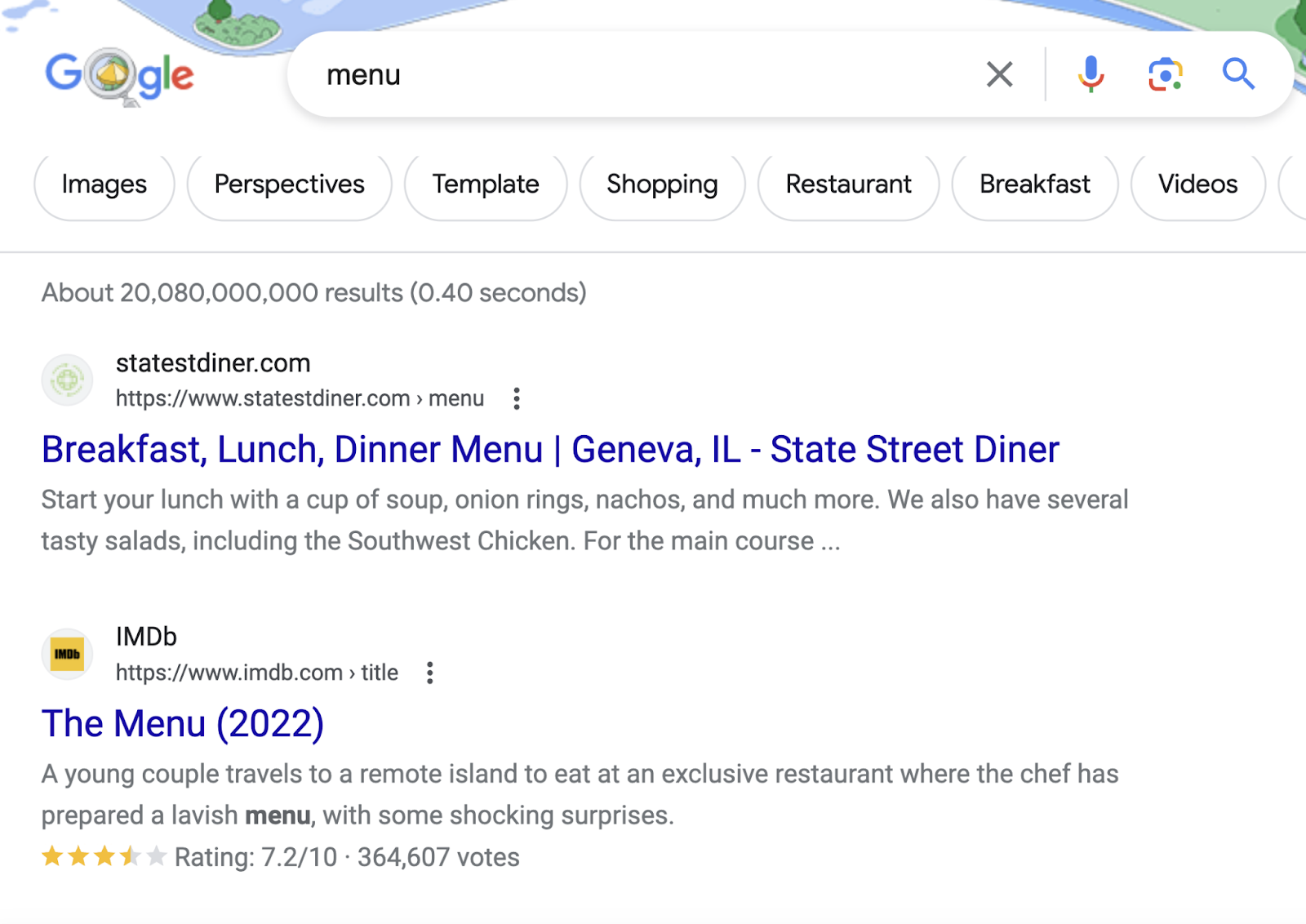**Detailed Caption:**

The image is a screenshot of a Google search page. At the top, the partially spelled logo "Google" appears with only "G" and "O" followed by "G-L-E". The letter "O" seems to contain an illustration that resembles an umbrella, which is magnified and possibly encircled by a magnifying glass. The background behind the Google letters shows imagery of water with a tiny island and a tree on the left side, though the tree is cut off at the trunk.

The search query inputted is "menu." The results are sorted by categories including Images, Perspectives, Template, Shopping, Restaurant, Breakfast, and Videos. Below the search bar, Google indicates approximately 20 billion results found in 0.40 seconds.

The first search result is from statestdiner.com, mentioning breakfast, lunch, and dinner menus for State Street Diner located in Geneva, Illinois. The diner offers menu items like a cup of soup, onion rings, nachos, and several salads, highlighting the Southwest chicken salad.

The second result is from IMDb (www.imdb.com) for the title "The Menu" (2022). The film's brief description involves a young couple traveling to a remote island to dine at an exclusive restaurant where the chef has prepared a lavish menu containing shocking surprises. The movie has received a rating of 3.5 out of 5 stars, or 7.2 out of 10, with 364,607 votes.